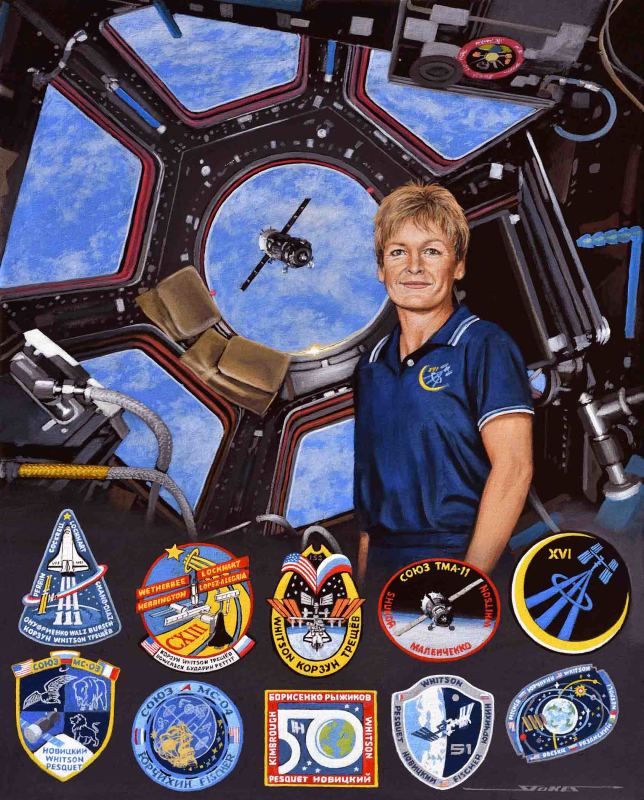This detailed image depicts an illustration of an older woman, possibly an astronaut, aboard the International Space Station (ISS). Positioned toward the middle right of the image, she has short blonde hair and is smiling. She is dressed in a blue polo shirt with striped accents on the sleeves and collar, along with blue pants. 

Above her, dominating the top portion of the image, is a prominent circular window of the ISS, outlined with trapezoidal panes through which a satellite and the Earth can be seen. 

Below this scene, the bottom third of the image is adorned with ten distinct space patches arranged in two rows of five. Each patch showcases a space-related theme, with one notable patch on the far left illustrating a rocket ship launching into space. The patches vary in shape, including circular, oval, and cone-like designs. The patches feature mixed languages, suggesting contributions from different countries.

Overall, the drawing vividly blends elements of space exploration, emphasizing the astronaut's role and international cooperation in space missions.